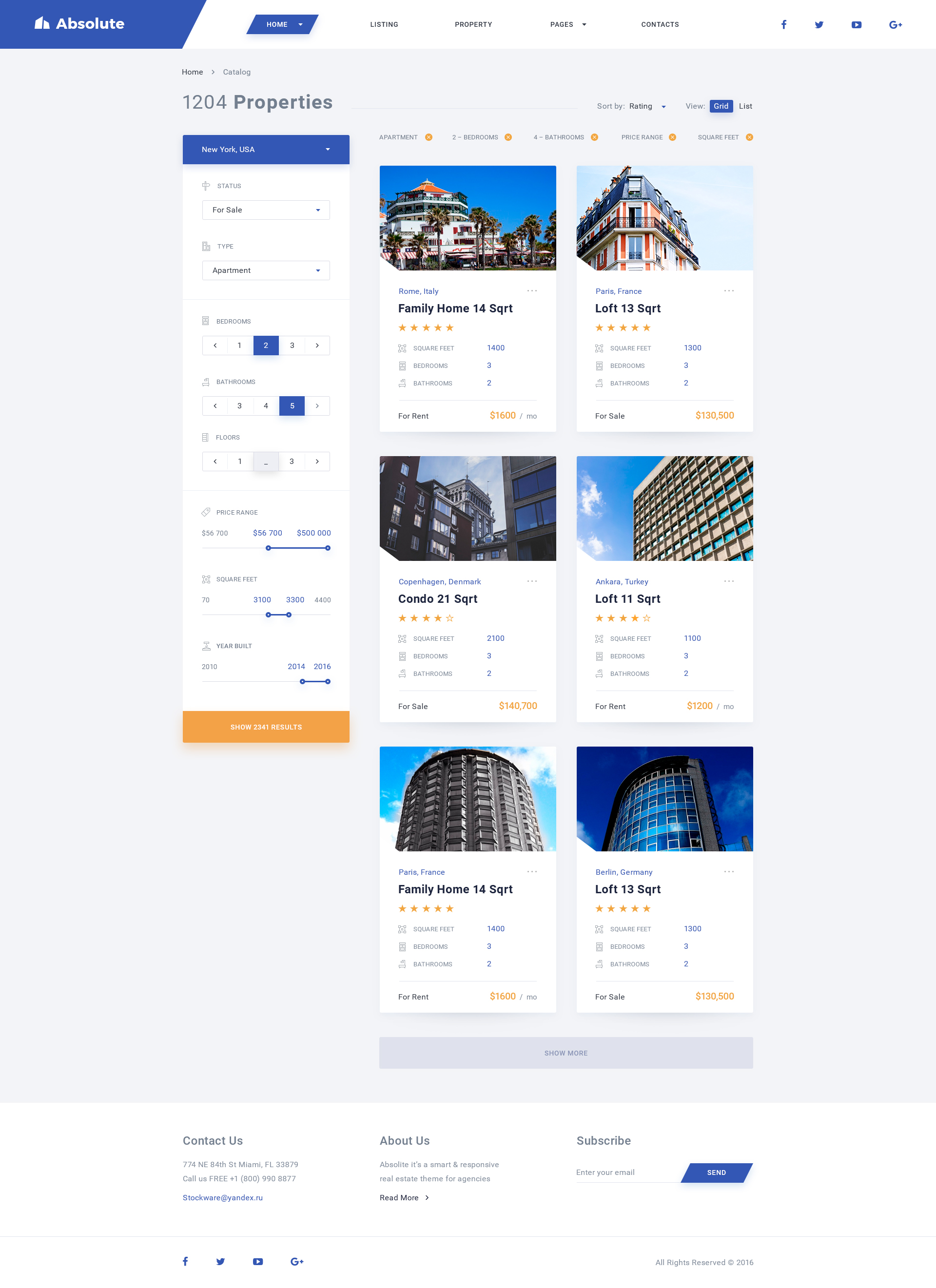The image features a web page with a sleek and organized design. In the top left corner, the word "Absolute" is prominently displayed in white text within a blue box. To its right, also in a blue box, is the word "Home." Adjacent to this, a few additional tabs are listed in black text on a white background, including "Listing," "Property Pages," and "Contacts."

In the top right corner, social media icons for Facebook, Twitter, YouTube, and Google Plus are visible. Below these icons, in gray text, is the total number of properties, noted as "1204 properties." Under this, within a blue area, the location "New York, USA" is displayed.

A white box below this area contains detailed filters for searching properties. These filters have drop-down menus for selecting options like "Status" (for sale), "Type" (apartment), "Bedroom" (with multiple options ranging from 1 to 12 selectable using left and right arrows), "Bathroom" (similarly navigable), and "Floors."

On the right side of the page, a few property listings are displayed in two columns with three items each. Each listing includes an image and a brief description. The listings are as follows:
1. "Family Home" with a size of 14 SQRT.
2. "Loft" with a size of 13 SQRT.
3. "Condo" with a size of 21 SQRT.
4. "Loft" with a size of 11 SQRT.
5. "Family Home" with a size of 14 SQRT.
6. "Loft" with a size of 13 SQRT.

Each property listing includes a thumbnail image, providing a visual preview of the respective property, and text descriptions below each image.